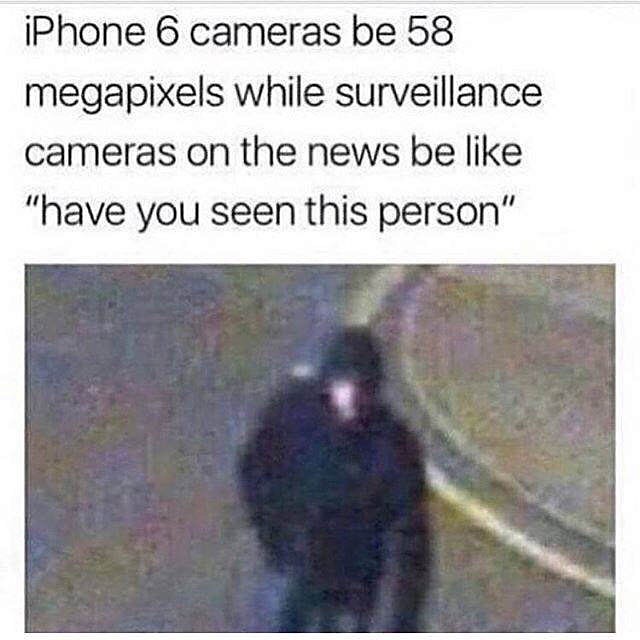The image is a meme contrasting the high-quality camera capabilities of an iPhone 6 with the low-resolution footage often seen from surveillance cameras. The top half of the image features black text on a white background that reads: "iPhone 6 cameras be 58 megapixels while surveillance cameras on the news be like, 'Have you seen this person?'". The bottom half of the image displays a heavily pixelated and blurry surveillance camera shot of a person standing on a concrete sidewalk, which appears slightly green and gray. The individual in the footage is wearing all dark clothing, including either a black hoodie or cap, and their face is a nondescript white blur. The lack of any discernible features renders the person unrecognizable, humorously suggesting the inadequacy of surveillance camera quality compared to modern smartphone cameras. The image also shows some pixelation and degradation around the text, emphasizing the poor quality of the surveillance footage.